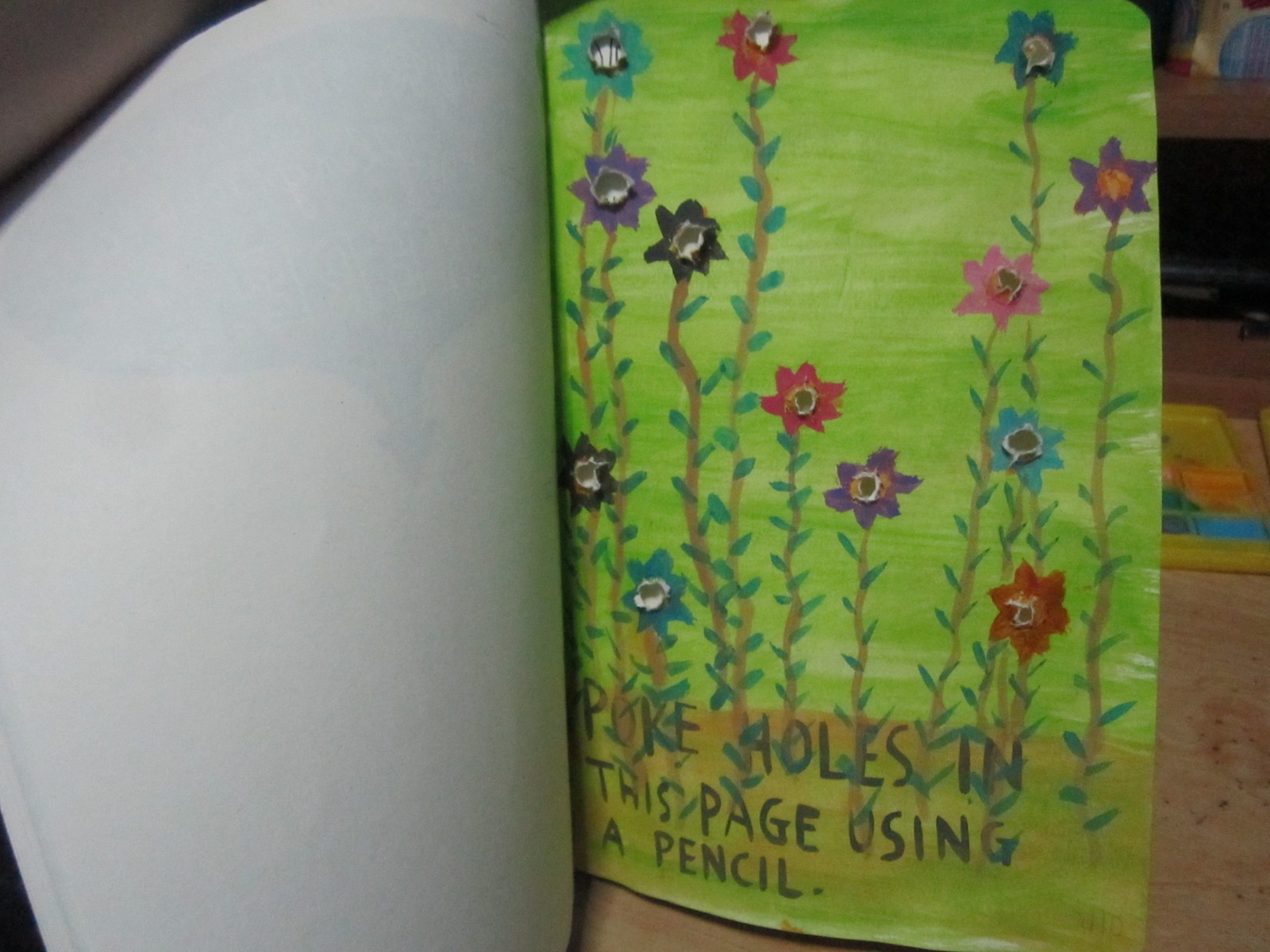The image depicts an open notebook or sketchbook with two visible pages. The left page is entirely blank, while the right page features a child's watercolor painting. The painting showcases a lush green background with a brownish-green area at the bottom, representing the ground. Rising from this base are numerous tall flower stalks, each adorned with small green leaves. Atop these brown stems are brightly colored flower petals in shades of red, blue, pink, violet, and teal. The middle of each flower blossom is punctured with holes, as per a handwritten instruction at the bottom of the page, which reads in capital letters: "POKE HOLES IN THIS PAGE USING A PENCIL." Adjacent to this watercolor piece, angled slightly, is a plain white piece of paper. The entire setup is placed on a brown surface, possibly a desk.